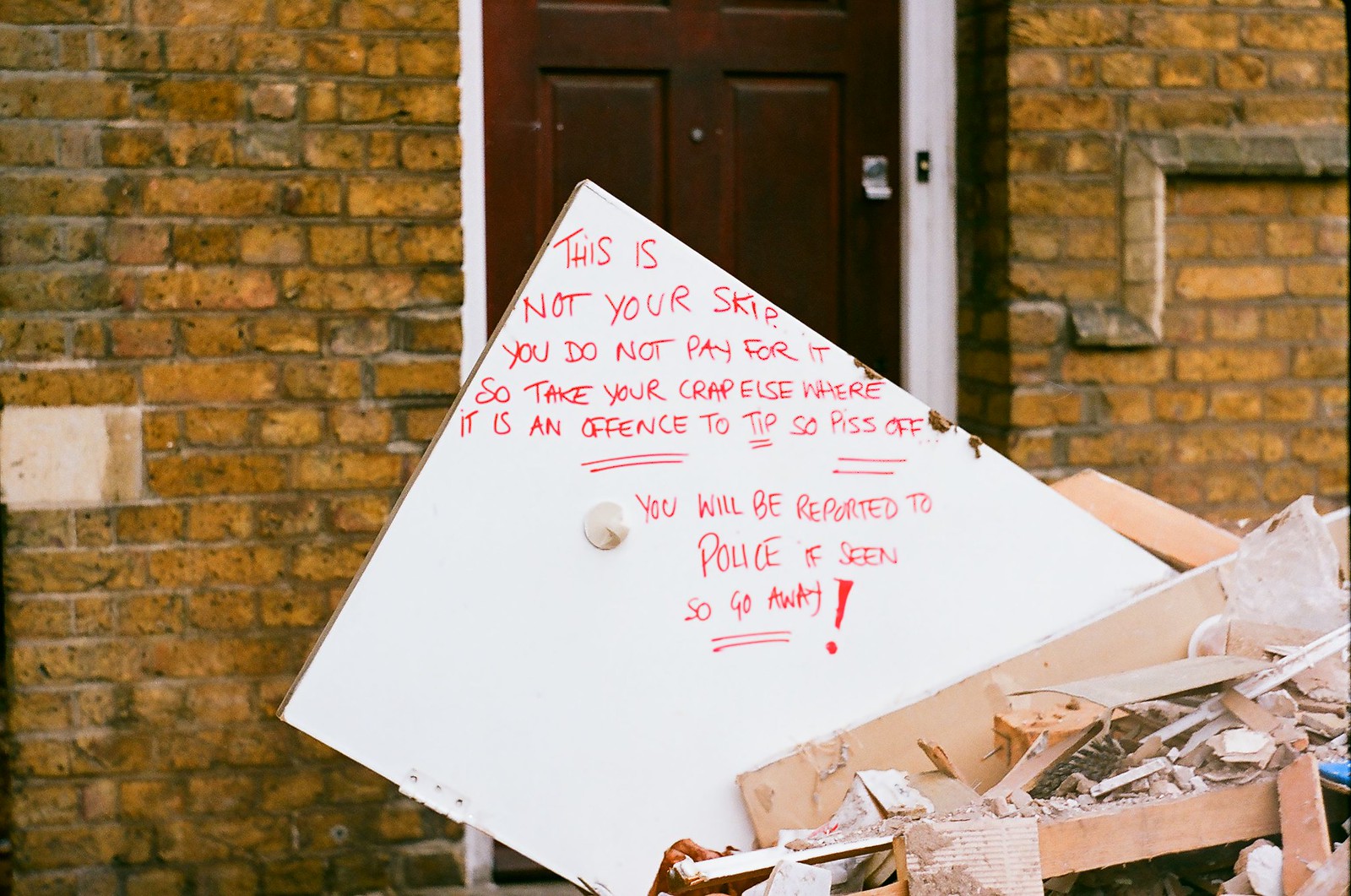The image depicts an outdoor scene in front of a brick building, which appears to be an apartment or house. At the center of the photograph is a dark brown wooden door, framed in white, set within yellowish, dirty brick walls. In front of this door lies a chaotic pile of building debris, including wood with nails, broken tiles, and other rubbish. Prominently sticking out from this rubble is a large white door, apparently torn off a building, tilted on its side. Written in red letters across the white door is an emphatic message: "This is not your skip. You do not pay for it, so take your crap elsewhere. It is an offense to tip, so piss off." Specific phrases such as "offense," "tip," "piss off," and "go away" are intensely underlined, and a giant red exclamation mark accentuates the message; the concluding lines warn violators that they "will be reported to the police if seen." The forceful language and multiple underlines convey a strong sense of frustration and urgency, commanding unauthorized dumpers to vacate the premises.